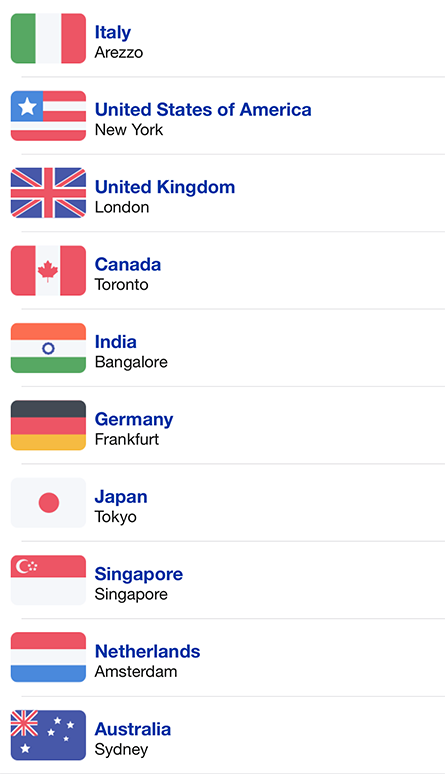This image displays a detailed list of countries, their flags, and major cities within those countries. The list is organized vertically and includes:

1. **Italy**
   - Followed by the Italian flag and the major city.
   
2. **United States of America** 
   - With the American flag and the city **New York** listed.
   
3. **United Kingdom**
   - Accompanied by the British flag and the city **London**.

4. **Canada**
   - Featuring the Canadian flag with **Toronto** listed as the major city.

5. **India**
   - The Indian flag with the city **Bangalore**, spelled as B-A-N-G-A-L-O-R-E.

6. **Germany**
   - Featuring the German flag and the city **Frankfurt**.

7. **Japan**
   - Including the Japanese flag and the city **Tokyo**.

8. **Singapore**
   - Represented with the Singaporean flag.

9. **Netherlands**
   - Accompanied by the Dutch flag and the city **Amsterdam**.

10. **Australia**
    - Displaying the Australian flag with the city **Sydney**.
  
Each country is represented at the top in bold, prominent font, followed by its respective flag. The corresponding city is listed directly below the country's name in a smaller, black font.